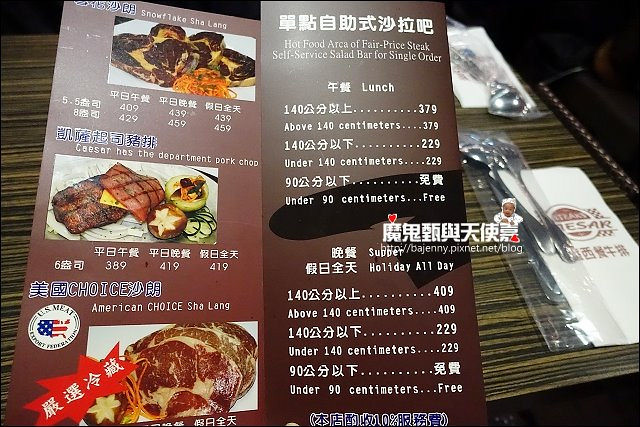The image depicts a blog post from the website http://bajeni.pixnet.net/blog. The blog features a distinct logo at the top, characterized by Japanese lettering adorned with hearts on the first and last characters. Beneath the logo, there's an image showing a baby dressed in a chef's uniform. The central focus of the blog post is a photograph of a restaurant menu placed on a wooden table.

In the photograph, the menu is partially folded, revealing a combination of Japanese and English (occasionally referred to as "Ingress") text. A white napkin features the word "Caesar," accompanied by additional Japanese characters. The table setting includes wrapped silverware, comprising a spoon and several forks.

The left side of the menu showcases images of various dishes, primarily focused on meats. One can observe a U.S. Meat Export Federation sticker towards the bottom left. The dishes displayed range from what appear to be meat-topped pretzels, chopped cooked ham, to bread wrapped in meat. 

The right side of the menu lists prices and descriptions. The limited English text indicates options like "Hot Food Area," "fair price steak," and "self-service salad bar for single order." Prices vary with size, such as 90 centimeters and below being free, and above 140 centimeters costing $3.79. The currency is unspecified. Additional pricing details for supper and holidays follow a similar pattern, with 90 centimeters free and above 140 centimeters priced at $4.09.

In summary, the blog post captures a detailed snapshot of a restaurant dining experience, emphasizing the menu and its offerings, alongside the author's personal website branding.